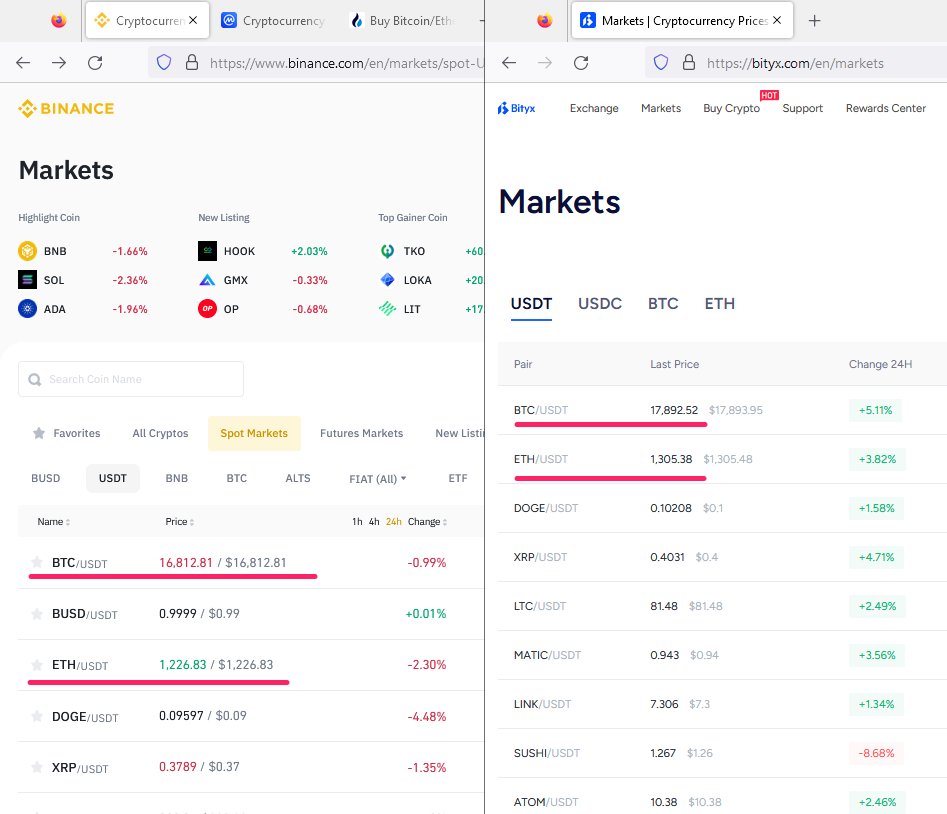The image displays two distinct screens featuring cryptocurrency market data. The first screen is labeled "Finance Markets" and lists nine different market categories, some showing negative percentages in red and others showing positive percentages in green. It includes sections labeled "Favorites," "All Crypto," "Spot Markets," and "Future Markets," each accompanied by a star icon. Below these headings, the screen lists five specific cryptocurrencies, providing detailed information on their names, current prices, and recent changes in value.

The second screen is titled "Bits Market" and includes sections for "Exchange Markets" and "Buy Crypto Markets." This screen showcases three distinct market categories, with two specific cryptocurrencies—identified as Bitcoin and Ethereum (ETH)—highlighted with a red line underneath them, indicating a decrease or potentially critical information. This layout provides a comprehensive overview of selected cryptocurrencies and their market performance.